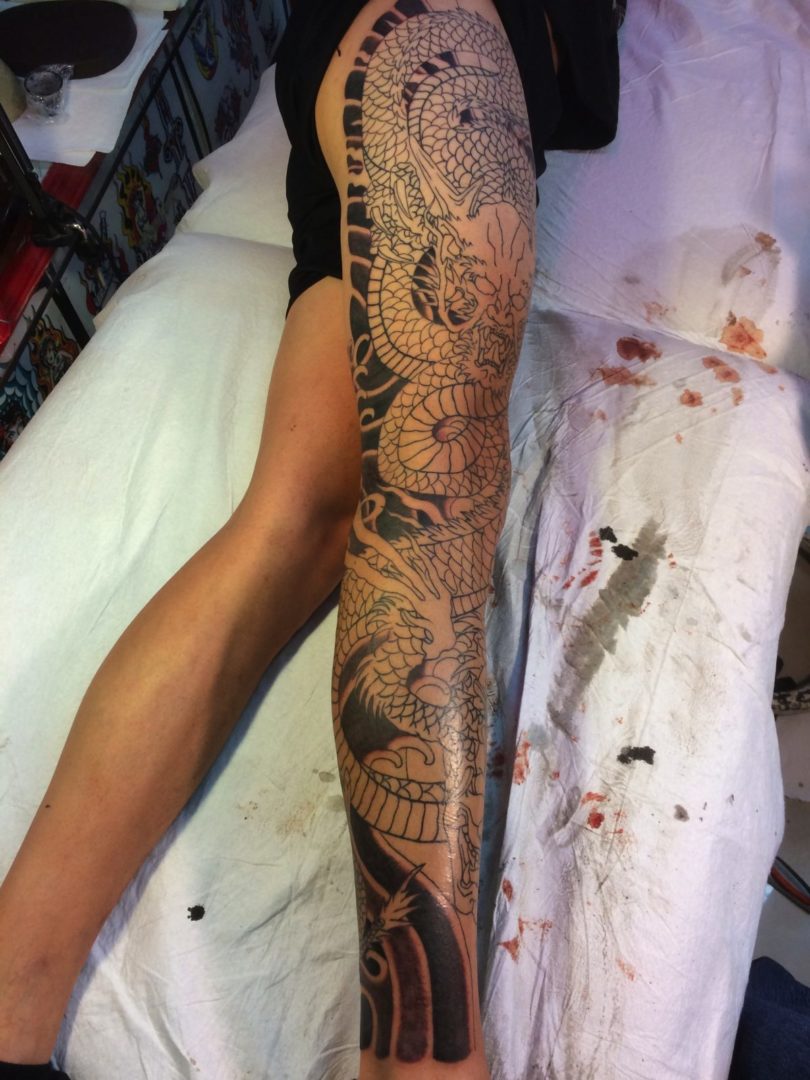The image depicts a man's legs positioned against a white sheet adorned with patterns of reddish, orange, and pinkish flowers, with accompanying leaves and stalks. His right leg, prominently featured, showcases an extensive tattoo that spans from his ankle to his hip. The tattoo, which has an intricate Hawaiian style, includes a dragon or snake-like design coiling up the leg in addition to a series of black bands, one extending from the buttocks to behind the knee and three more near the ankle. In stark contrast, his left leg is completely bare, devoid of any tattoos or patterns. The setting is somewhat ambiguous, with an unclear structure behind him, possibly a stained-glass surface or another textured material. Notably, there are splotches of blood on the right-hand side of the sheet, hinting at the recent and potentially painful completion of the tattoo.